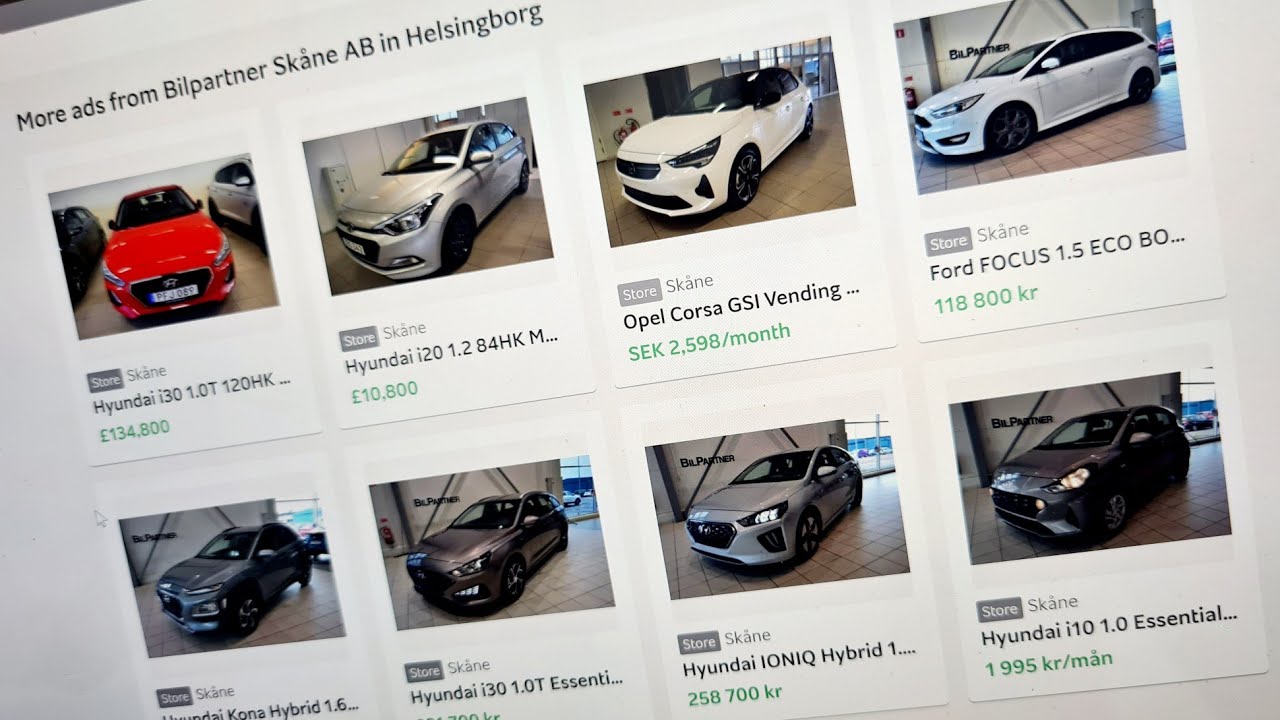This image captures the storefront of an automobile dealer's website, featuring a variety of cars available for sale under the banner of "More ads from PhilPartner," located in Skåne, AB, and Helsingborg. It showcases eight different automobiles, each with specific details and prices.

1. **Hyundai i30 1.0T 120HK** - A vibrant red compact car priced at £134,800.
2. **Hyundai i20 1.2 84HKM** - A sleek white SUV available for £10,800.
3. **Opel Corsa GSI Vending** - Featured with a monthly installment option of £25.98, highlighting its affordability.
4. **Ford Focus 1.5 EcoBoost** - Priced at £118,800, this car combines efficiency and modern design.
5. **Hyundai Kona Hybrid 1.6** - A stylish black SUV, although part of the description is cut off.
6. **Hyundai i30 1.0T Essential** - The price for this model is not fully visible.
7. **Hyundai Ioniq Hybrid 1** - A grey SUV priced at £258,700, blending hybrid technology with practicality.
8. **Hyundai i10 1.0 Essential** - Available at £1,995 per month, marked as an essential and economical choice.

Each vehicle is clearly advertised with the dealer's name, Skåne, in the picture descriptions, providing potential buyers with a comprehensive overview of their options.